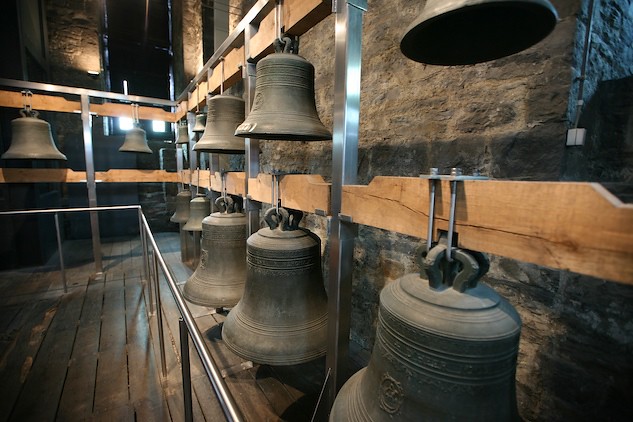The image is a color photograph taken inside an old, historical landmark, possibly a clock tower or church building. The scene is slightly dark, but well-lit with both artificial lighting and sunlight streaming through windows in the background. Stone walls envelop the space, adding to the historic feel, and the floor is made of old wooden floorboards. Central to the image are several large, antique bells, hanging in two layers from wooden boards shaped like a trapezoid. These bells appear to be made of patinaed metal, giving them a dull, grayish look reminiscent of old bronze or iron. A metal railing secures the area, preventing access to the bells, which seem to be part of a display. The image, captured at a diagonal angle, shows the closest bell to the right and the furthest bell to the left, creating a dynamic perspective of this evocative and meticulously preserved historical setting.